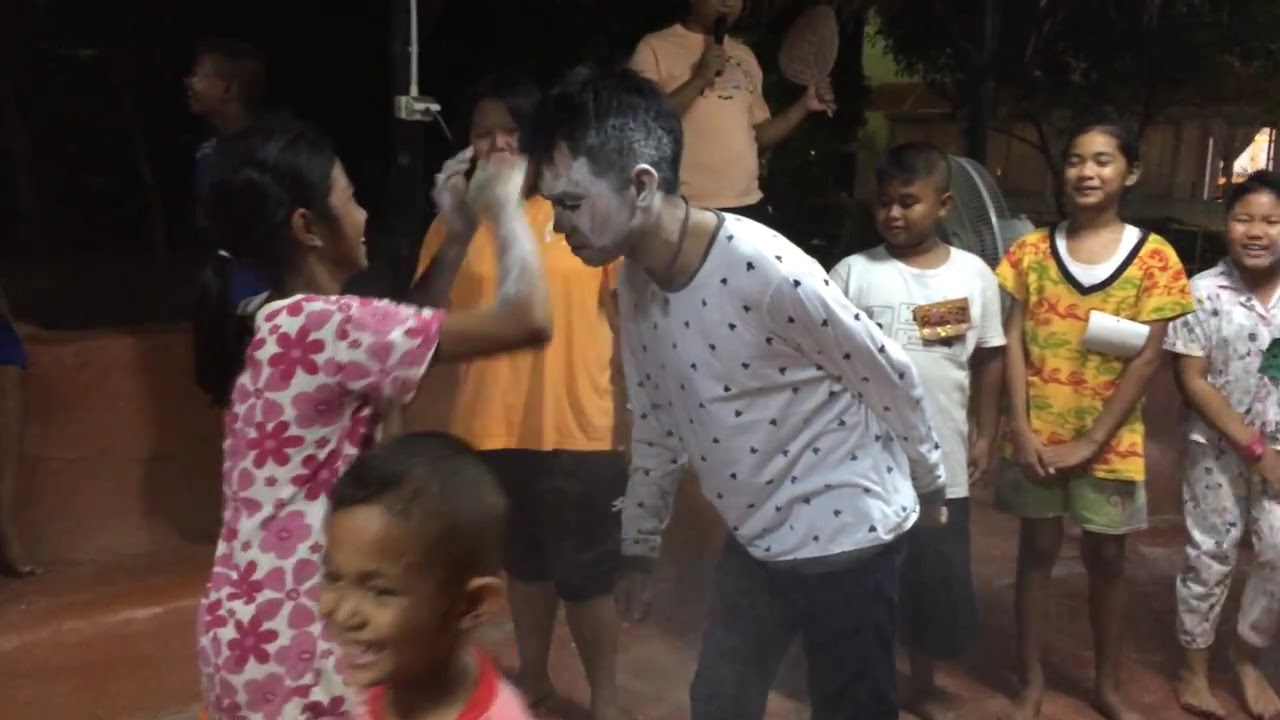In this outdoor evening scene, about half a dozen children, aged between 5 and 10, are gathered in a semi-circle, joyfully observing two central figures—a girl and a boy. The girl, of Asian descent with brown skin and black hair tied in a ponytail, is wearing a white shirt adorned with pink flowers. Her hands and forearms are raised, covered in a white, chalky substance, possibly resembling the traditional face powder used in Myanmar. She appears to be smearing this substance onto the boy standing in front of her. The boy, whose black hair and face are dusted with the same white substance, is leaning forward with his eyes closed. He wears a white long-sleeved shirt with fine blue dots and black pants. Off in the background, children in regular street clothes are laughing and enjoying the playful scene. An adult, visible from the lower face to the mid-waist and clothed in a white shirt, stands centrally. He holds a cordless microphone in his right hand and a hand fan in his left, looking down at the children. A prominently featured boy in the foreground, smiling widely, adds to the joyful atmosphere as he runs around, surrounded by laughter and celebration.